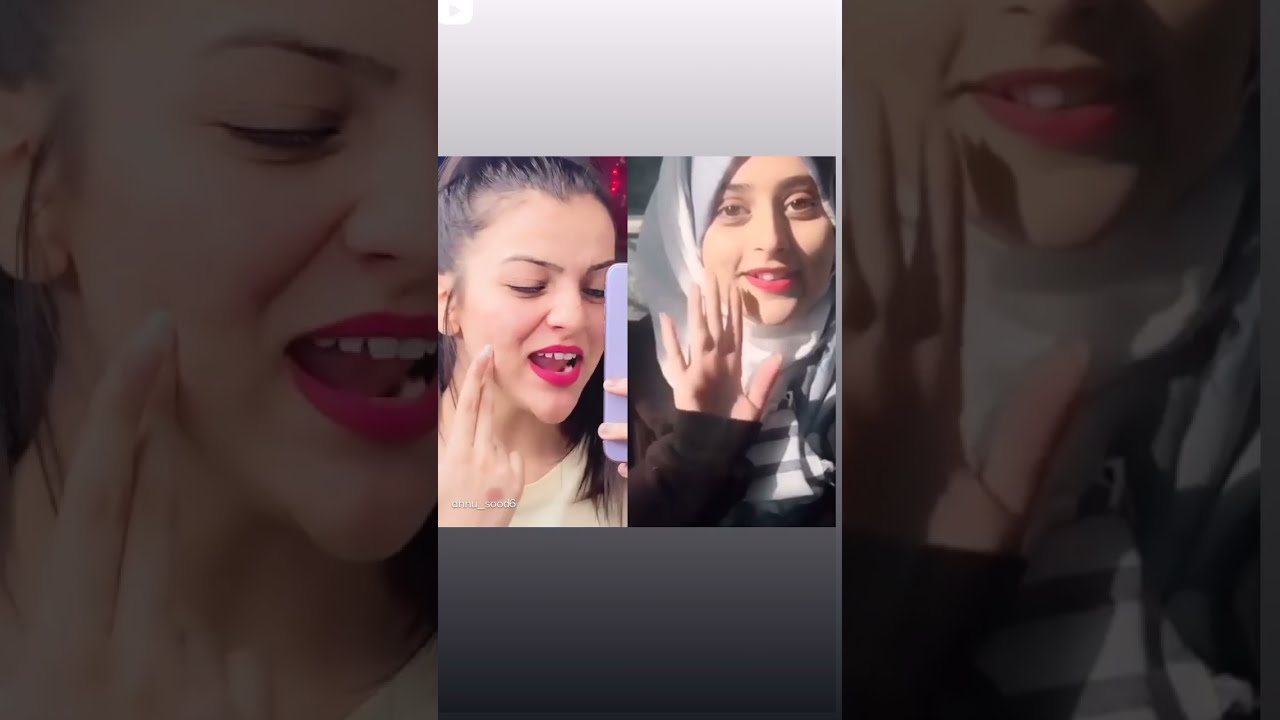This image is a screen grab from a video, showcasing a split-screen format with two young women. On the left side, the woman has long dark hair slicked back, and is seen wearing a yellow blouse, while holding a cell phone with a lavender case. She has pink lipstick on and is applying makeup to her cheek with one finger, her mouth open as if speaking or explaining something, likely related to makeup. On the right side, the second young woman wears a headscarf and has pink lipstick. She is depicted with her right hand raised, either in a waving gesture or a signal to not take her picture. She wears a black sweatshirt with a striped shirt or scarf underneath. This looks like a makeup discussion video, possibly on YouTube, as indicated by a faint YouTube logo on the top left corner of the light gray background.